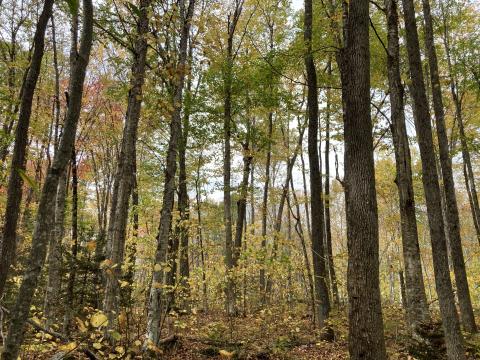This is a color photograph taken during daytime in a sparse, autumnal forest. The image captures a variety of tall, slender tree trunks, predominantly grouped on the left and right sides of the frame, creating an open space in the middle. The trees, ranging from thin to occasionally thick trunks, reach high into an overcast sky that reveals patches of blue. Toward the top of the trees, leaves are primarily green, while the lower foliage displays vibrant yellow and red hues, indicative of the fall season. The forest floor is covered in brown, dried leaves that have fallen, adding to the autumnal atmosphere. The setting is not dense, allowing ample light to filter through, and in the background, a clearing can be seen that gives a sense of openness and additional light to the scene. Scattered evergreen trees contribute flecks of green among the more prevalent turning leaves. Overall, the photograph portrays a serene, lightly wooded area bathed in the soft, diffused light of an autumn day.